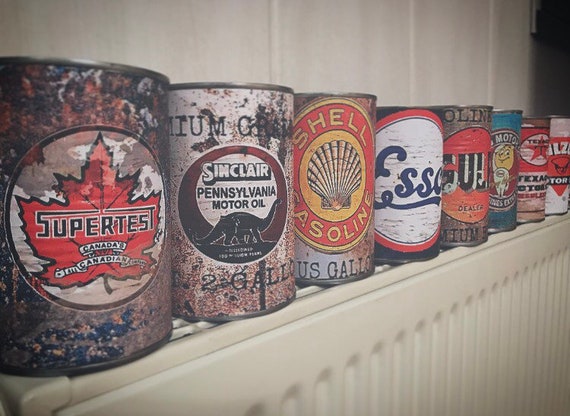The photograph captures a shelf adorned with a collection of eight colorful, vintage metal cans, possibly made of aluminum or steel. Arranged on a white shelf, each can boasts distinct designs and branding, offering a nostalgic glimpse into various products from the past. To the far left stands a grayish can labeled "Super Test," featuring a prominent red maple leaf and the words "Canada" and "Canadian." Next to it, a white and brown can showcases a dinosaur and the inscription "Sinclair Pennsylvania Motor Oil," its appearance weathered with age and wear. Following this, a Shell gasoline can catches the eye with its yellow, red, and gray hues and a central seashell image. Adjacent to it is an Esso can, characterized by a white, red, and dark blue color scheme and blue cursive lettering. The lineup continues with a golden and red can, a blue can, and a red can with a star in the center. Concluding the array is a white and red can. These tins, likely vintage oil cans, are meticulously aligned, creating a visually compelling display that reflects a bygone era.